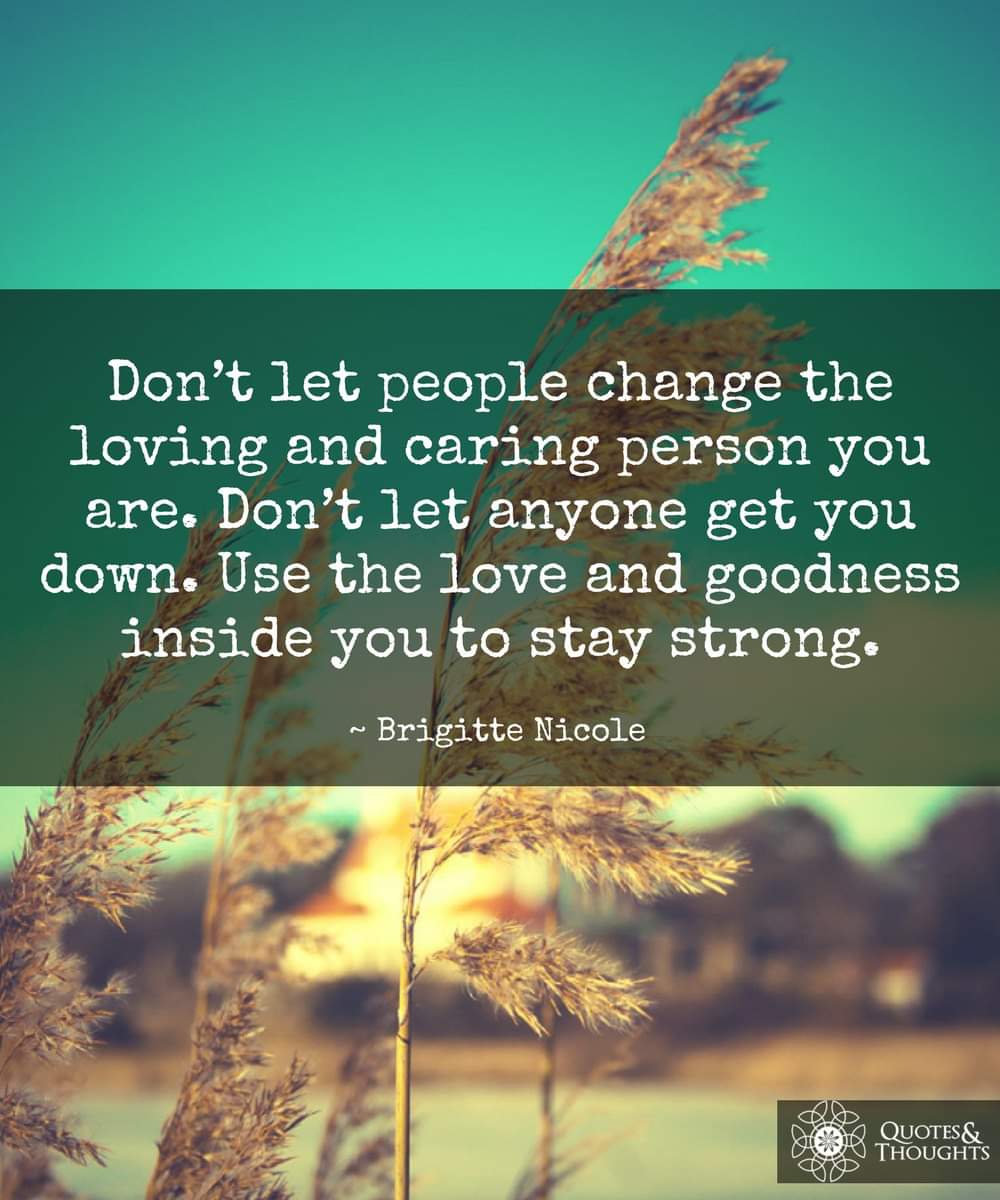The image features a serene, bluish-green background with faintly visible wheat or brownish branches of a tree or plant, suggesting an outdoor scene. Superimposed on this backdrop is a translucent black overlay bearing a quotation in white text. The quote, "Don't let people change the loving and caring person you are. Don't let anyone get you down. Use the love and goodness inside you to stay strong," is attributed to Bridget Nicole and is centrally placed across the middle of the page. At the bottom right-hand corner, another translucent black rectangle contains the words "quotes and thoughts" next to a symbolic white circle with an intricate flower pattern radiating outward. The overall design is calm and meditative, accentuated by the soft, faded appearance of the background elements.